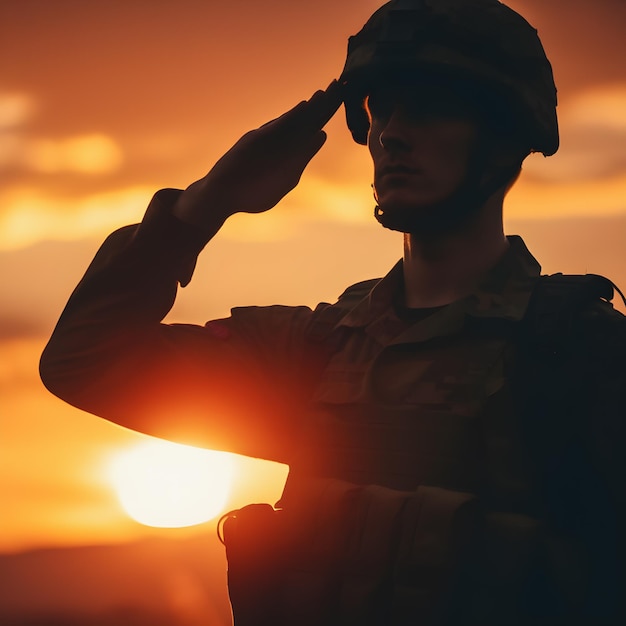This photograph captures a young soldier, likely between the ages of 18 and 25, saluting with his right hand against a stunning sunset backdrop. The soldier is adorned in full camouflage military uniform, including a helmet securely fastened under his jaw. Though the image is primarily silhouetted, the pale complexion and distinct facial features such as his long jawline and pointed nose are faintly perceptible. The scene is dramatically lit by the sunset, which casts a golden, yellow, and orange glow across the sky. The sun peeks from below the soldier’s raised elbow, further accentuating the silhouette effect. The focus is sharply on the soldier, who occupies three-quarters of the photo from the waist up, with the sky in the background appearing blurry. The overall ambiance evokes a sense of solemn commitment, as the soldier looks westward, his facial expression serious and his mouth firmly closed, embodying the dedication and resolve of military service.